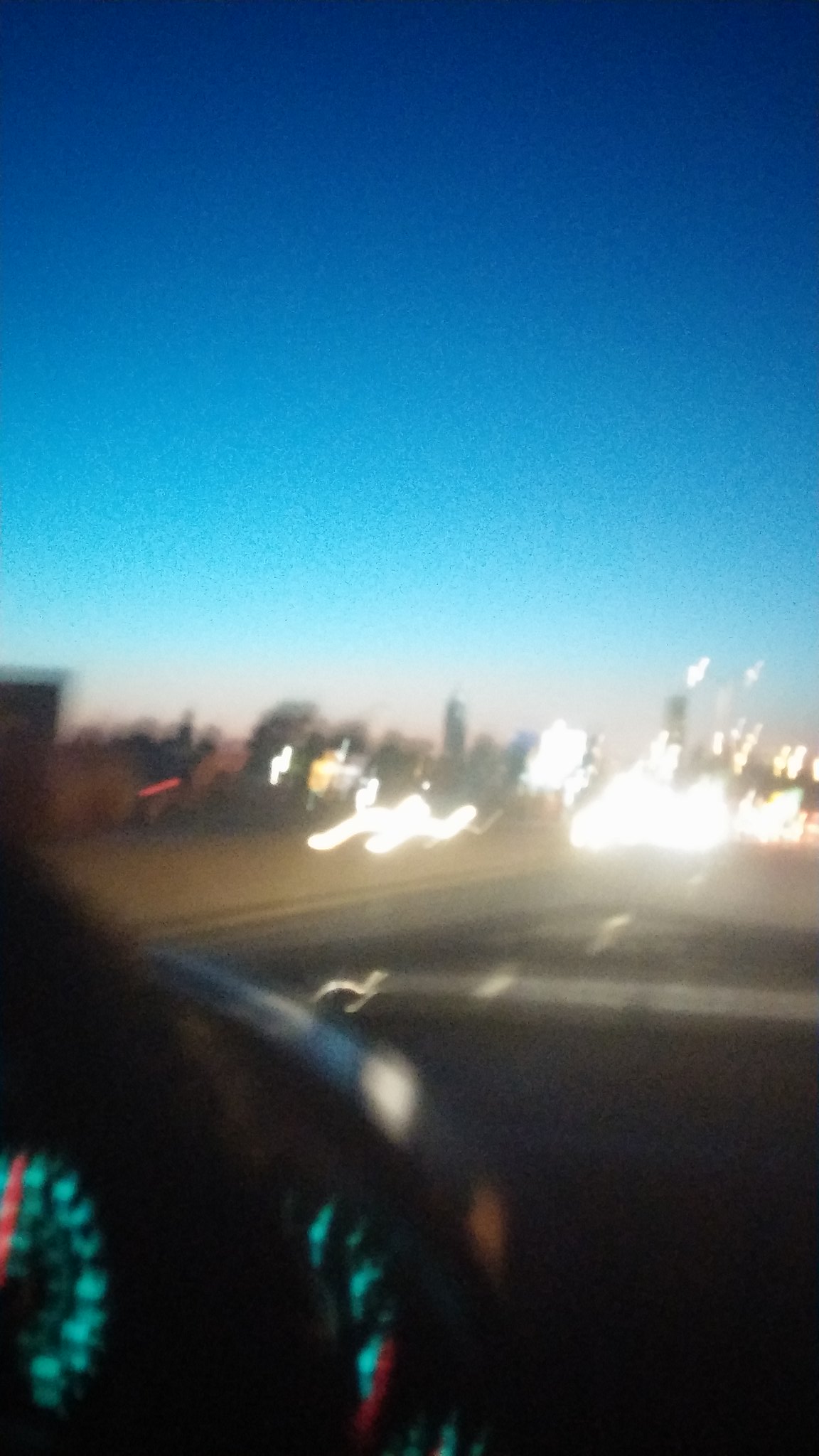The photograph captures an early morning view from inside a moving car on a bustling highway. Taken by the driver, the image is slightly blurry, indicating motion. The black steering wheel and illuminated speedometer are visible, bathed in a green light. Out through the windshield, the cityscape comes into view with silhouettes of buildings and trees under a pre-dawn sky that transitions from dark blue at the top to a gradient of light blue and orange near the horizon. The highway ahead is crowded with vehicles, their headlights creating a blur of bright lights, contributing to the busy atmosphere. Despite the blurriness, the image conveys the energy of a city just waking up as daylight begins to break.